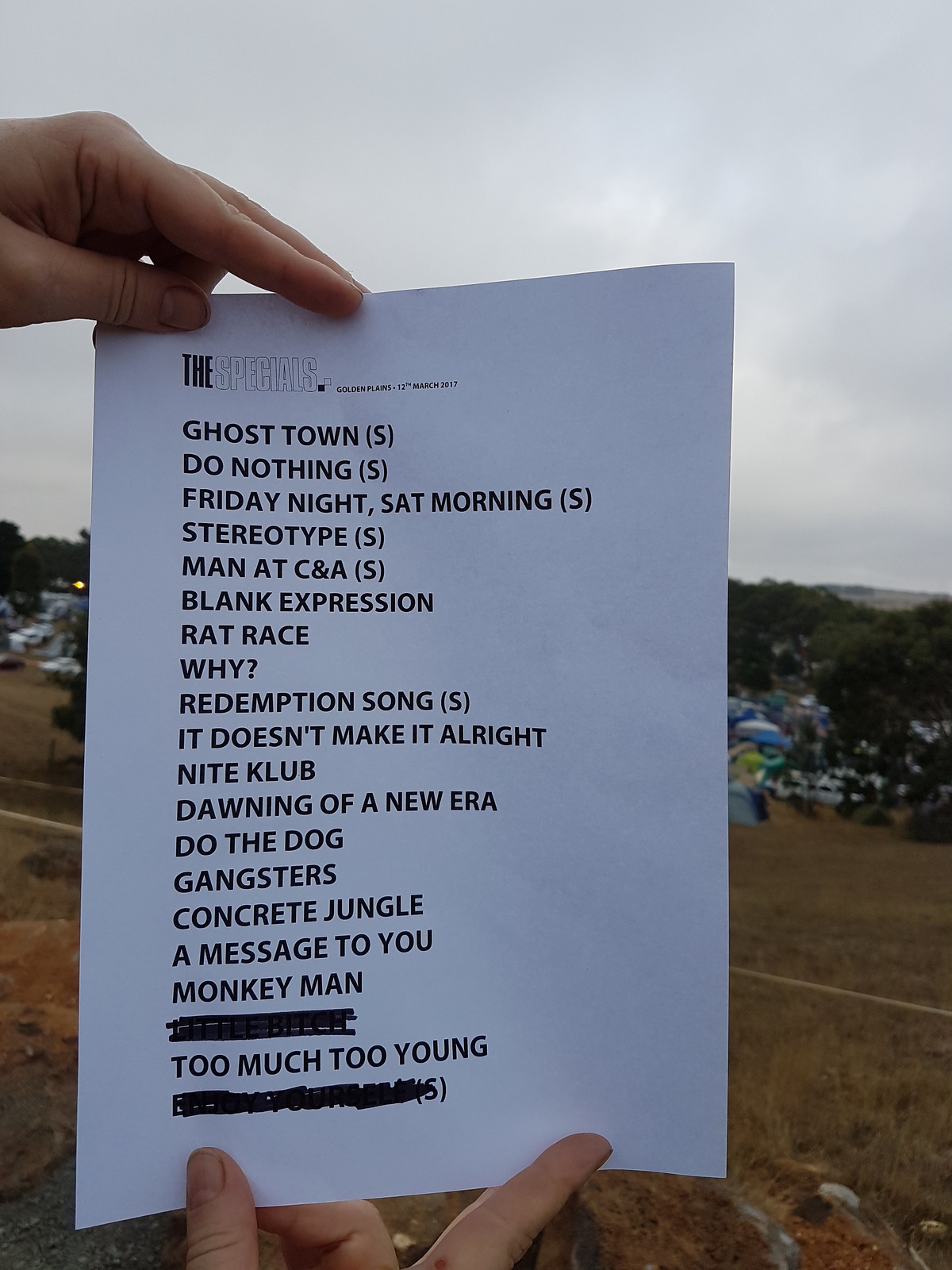The photograph depicts an outdoor festival scene with a hilly area blanketed in brown and beige grass leading down to a bustling area filled with numerous tents, cars, and lush green trees. Overhead, the sky is overcast with light gray clouds. In the foreground, prominently highlighted, two white hands hold up a white printed piece of paper towards the camera, their presence dominant in the image. The piece of paper, seemingly a set list for a band named "The Specials," is emblazoned with the band's logo at the top. Below, in smaller black text, it states "Golden Plains, 12th March 2017." The song list starts with titles like "Ghost Town," "Do Nothing," "Friday Night, Saturday Morning," "Stereotype," "Man at C&A," "Blank Expression," "Rat Race," "Why," "Redemption Song," "It Doesn't Make It Alright," "Nightclub," "Dawning of a New Era," "Do the Dog," "Gangsters," "Concrete Jungle," "A Message to You," "Monkey Man." Notably, two songs, "Too Much Too Young" and another at the bottom, are crossed out. Only the hands holding the paper are visible, the left hand gripping the top edge, and the right hand supporting the bottom of the sheet, emphasizing the paper against the contrasting festival scene in the background.